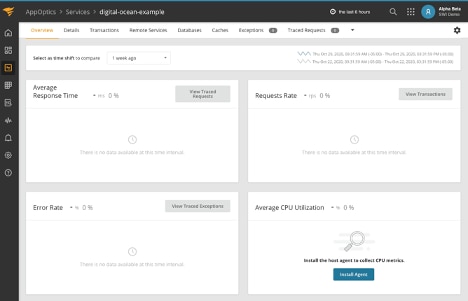This screenshot showcases a back-end page within the settings menu of a software application, specifically for AppOptics services integrated with DigitalOcean, as indicated by the heading "AppOptics Services Digital Ocean Example" at the top of the page. The layout features a narrow black sidebar on the left, adorned with various icons, and a prominent yellow icon positioned at the top left corner. On the top right corner of the interface, there is a blue circular icon. The main content area is divided into four large, white sections: "Average Response Time" occupies the top left, "Request Rate" is to the top right, "Error Rate" is located at the bottom left, and "Average CPU Utilization" is positioned at the bottom right. This structured setup allows for streamlined monitoring and management of key performance metrics for the application’s performance on DigitalOcean through AppOptics services.